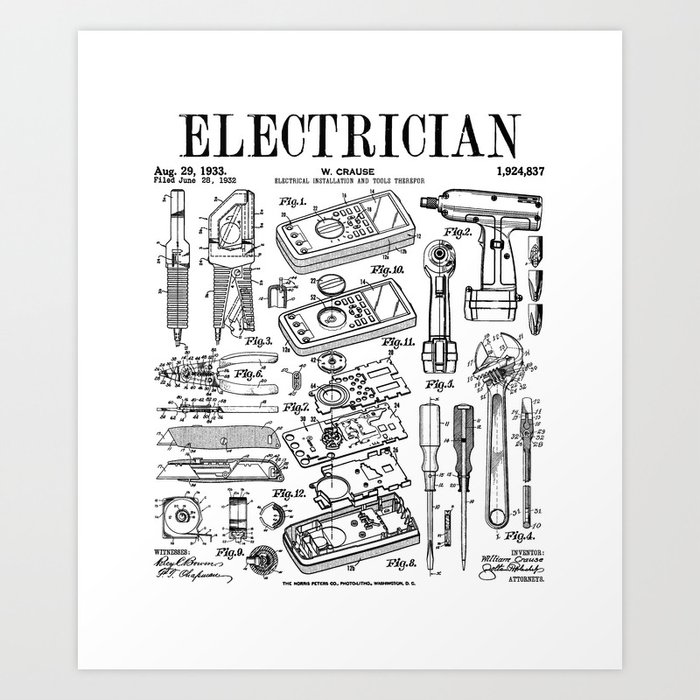This image is a detailed black-and-white informational poster titled "ELECTRICIAN" in bold black capital letters at the top. It is divided into three columns with the following headings: August 29, 1933, W.C.R.A.U.S.E., and the number 1,924,837. Each column features various technical drawings and diagrams of electrician's tools.

Under the heading August 29, 1933, the poster shows illustrated tools, including an electric screwdriver, a regular screwdriver, a wrench, a knife, wire cutters, clippers, and a tape measure, along with additional pieces and knobs. Small, faint black writing appears at the bottom of this column.

The middle column under W.C.R.A.U.S.E. displays what appears to be the intricate details of an electrical installation, dissected parts of an instrument or gauge, highlighting its inner workings through progressive diagrams. This column also has small, barely legible writing at the bottom.

On the right side, under the number 1,924,837, there are drawings of an electric drill from different angles – a profile and a front view. Below the drill, there are more illustrations of screwdrivers, a wrench, and clippers. Figures highlighted include numbers 4, 7, 8, 9, 11, and 12, with a small amount of faint text at the bottom right corner of the column.

The entire poster appears to be set against a light gray background, emphasizing the intricate black-and-white details of the technical equipment displayed.